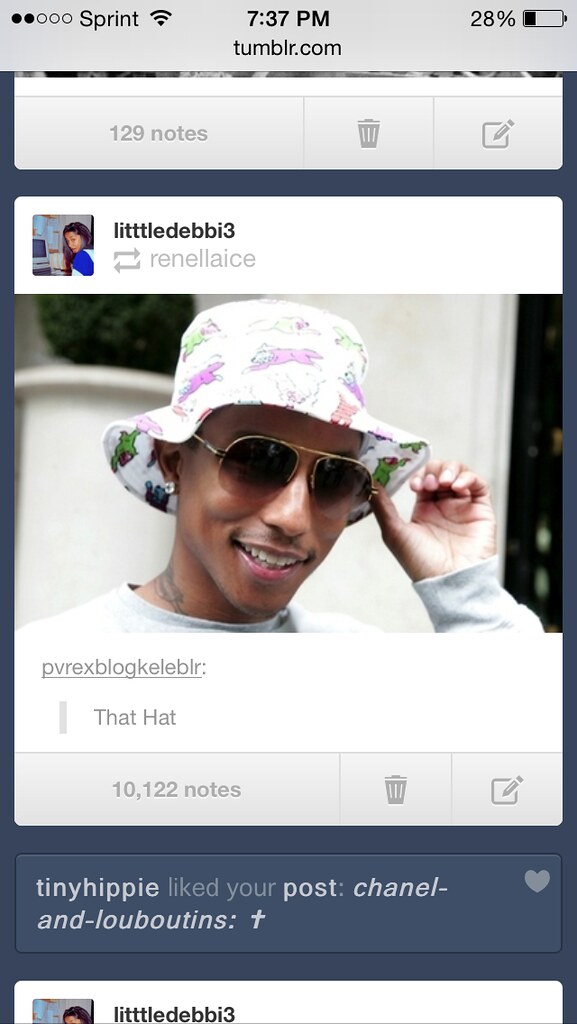This detailed image is a tall, rectangular screenshot taken from an iPhone displaying a Tumblr post. The top bar indicates the carrier as Sprint, the time as 7:37 PM, and the remaining battery at 28%. It shows the URL as tumblr.com and indicates that the post has 129 notes. 

The main content features a post re-shared by Little Debbie 3, originally from username "R-E-N-E-L-L-I-E-A-I-C-E." The central image is a headshot of musical artist Pharrell Williams, wearing a white floppy hat with a colorful pattern of pink and green characters, dark aviator sunglasses, and a broad smile. He is posed center-frame, adjusting his hat with his left hand. 

Below the image, there's a gray banner noting "10,122 Notes" with a trash can (delete button) and a pencil icon (edit button) nearby. At the bottom of the screenshot is a navy-blue footer stating "Tiny Hippie Liked Your Post" with the text "Chanel and Louboutins" below it. 

The colors featured in the image include shades of gray, black, white, blue, brown, purple, green, and gold, emphasizing a blend of both site interface and visual content.